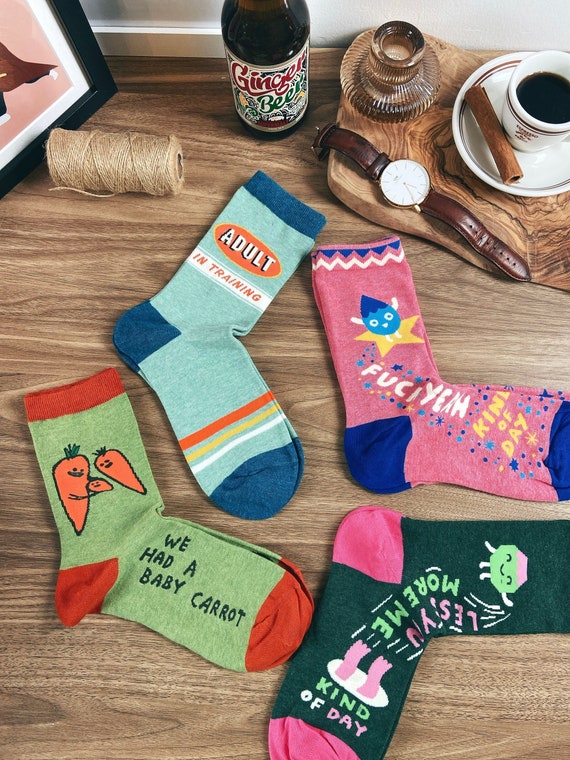In a portrait-oriented, aerial view photograph, a wooden table with prominent oak grain running horizontally serves as the backdrop. The lower two-thirds of the image feature four pairs of colorful socks laid out prominently. The left-most pair is vibrant with a green background, red heels, toes, and cuffs, adorned with animated carrot characters - one carrot holding a baby carrot, all with smiley faces, and the words "we had a baby carrot" embroidered on the sole in dark green. 

Adjacent to these are a pair of baby blue socks with dark accents and the text "adult in training." The third pair is primarily dark gray with pink tips and heels, featuring the text "less you, more me" and "fuck yeah kind of day" partially visible due to a slight fold. The fourth pair has a pink design with blue accents and reads, "if you see yeah, kind of day," also featuring a small character on a gold star.

In the upper part of the image, partially out of frame, are several items adding to the eclectic scene: a roll of twine in front of an indistinct photo frame, a glass brown bottle of ginger beer, and a rustic, uneven wooden plate. On this wooden plate rests a small white china espresso cup filled with dark coffee and garnished with a cinnamon stick, alongside a brown leather strap watch with a white clock face and gold hands. A ribbed glass jar and a glass quill-like object complete the assortment. The setting appears against a white wall, with the trim hinting the image was taken at floor level.